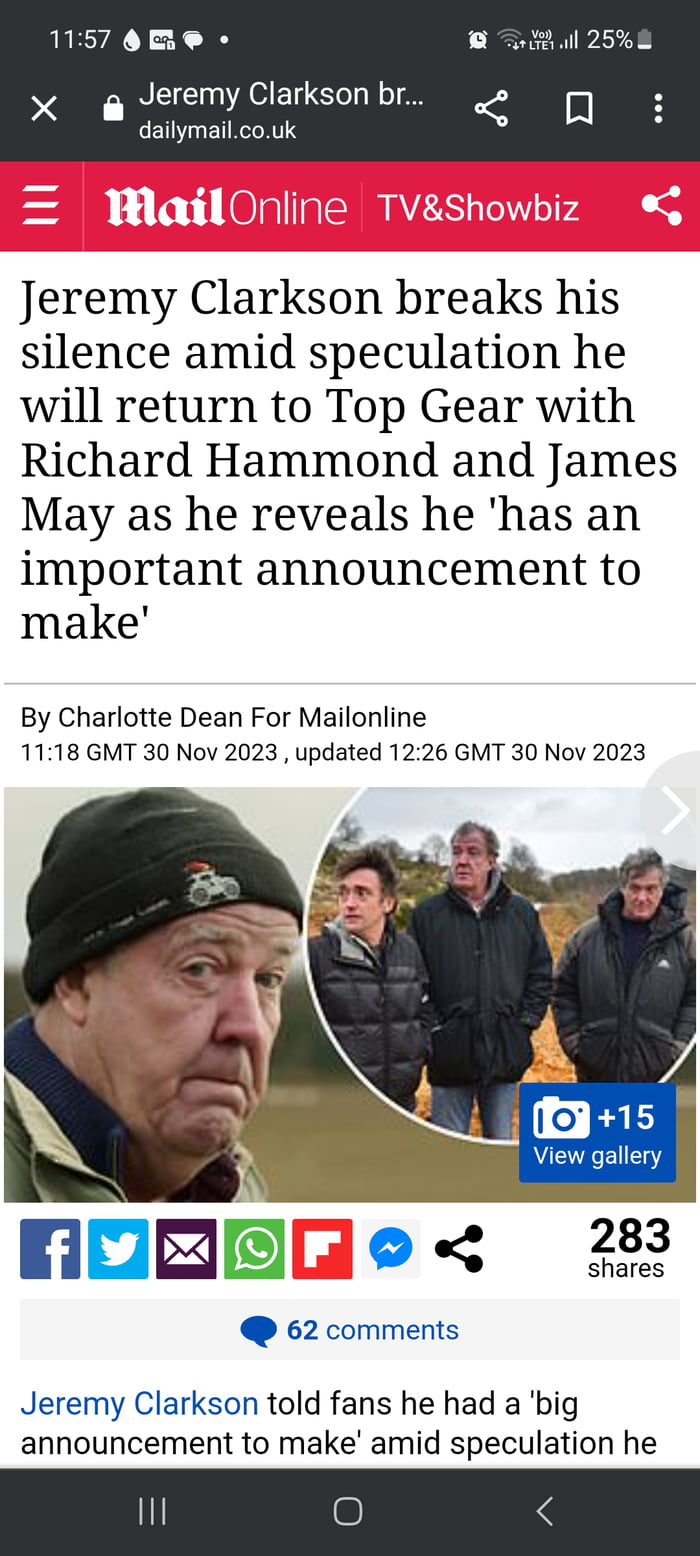A smartphone screen displaying an article from the Daily Mail UK is shown. The title reads, "Jeremy Clarkson Breaks His Silence Amid Speculation He Will Return to Top Gear with Richard Hammond and James May," authored by Charlotte Dean for Mail Online TV and Showbiz. The article mentions Clarkson has an important announcement. It was published at 11:18 GMT on 30 November 2023 and updated at 12:26 GMT on the same day. The article includes an inset circular image with three men, presumably Clarkson, Hammond, and May, all wearing black jackets and looking to the left. The main photograph shows an older man, likely Jeremy Clarkson, wearing a black stocking cap and looking doubtful. Additional indicators on the screen show a 25% phone battery, the time as 11:57, and signal bars. The article’s sidebar notes there are 15 more images to view in the gallery, alongside social media sharing options (Facebook, Twitter, Email, Facebook Messenger) and metrics indicating 283 shares and 62 comments.